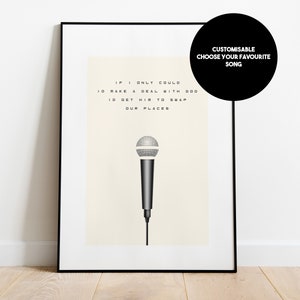This image is an advertisement for a customizable piece of art that features a framed portrait with a black border and a white mat. The centerpiece of the portrait is a digital graphic of a black microphone with a light gray top. Above the microphone, there are song lyrics typed in black font, although they are too small to read clearly. The background of the art piece is off-white, and it is sitting on a wood plank floor against a white wall, casting a shadow to the left. A black circle overlaying the microphone graphic bears the white text: "Customizable. Choose your favorite song." The overall scene suggests a modern and sleek design, perfect for personalizing with one's favorite song lyrics.